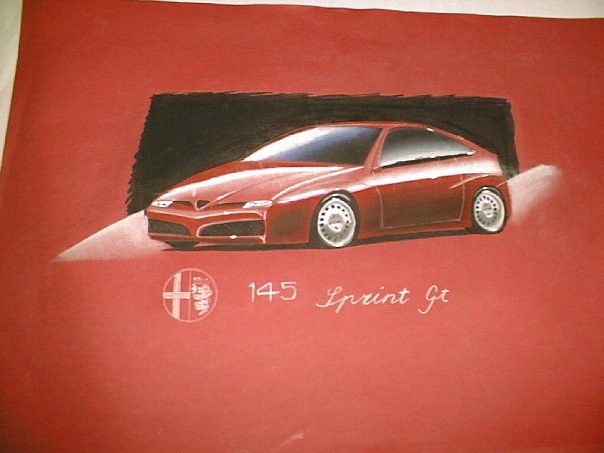The image appears to be a meticulously hand-created graphic that resembles an advertisement storyboard. Dominating the composition is a bold red background, slightly faded and discolored in certain areas to add a sense of texture and depth. Nestled centrally on this vibrant canvas is a sleek, sporty red car, poised in front of a subtle black square backdrop. The car boasts a dark-colored windshield that adds to its aerodynamic appeal, flanked by striking white headlights and a black grille below. Its black tires feature prominent silver hubs, enhancing the car’s polished aesthetic.

Illuminating the scene, there are bright white lights that emanate from both behind and in front of the car, accentuating its contours and highlighting its dynamic presence. Below the car, a distinctive white circle is visible. It contains a cross on one side and intricate squiggles on the other, both adding to the visual intrigue. Inscribed at the bottom of the image is a series of white alphanumeric characters, designed to catch the viewer's attention and perhaps provide additional information or branding context.

In summary, the image is of very high quality, exhibiting crisp lines and vivid details that combine to create a compelling visual narrative.